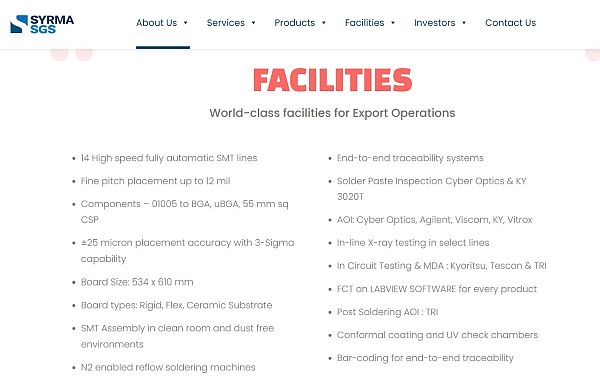Here is the cleaned-up and detailed caption for the image:

---

This image is from the website of a company named SYRMASGS. The layout consists of a black top section and a blue bottom section. Dominating the visual design are two uniquely shaped triangles that intersect. The website's main navigation menu includes options such as "About Us," "Services," "Products," "Facilities," "Investors," and "Contact Us," with "About Us" highlighted by an underline in black.

Central to the image is a bold red header stating "Facilities," featuring the slogan "World-Class Facilities for Export Operations." Beneath this header is a comprehensive list of facilities and features, organized with bullet points:

- 14 high-speed fully automatic SMT lines
- Fine pitch placement up to 12 mil components
- 25 micron placement accuracy for components
- Accommodates various board sizes and types
- SMT assembly and end-to-end reflow processes

On the right side, further details highlight advanced systems and equipment, such as:

- End-to-end traceability system
- Solder paste technology
- Automated Optical Inspection (AOI) by CyberOptics
- In-circuit testing
- Pass soldering capabilities
- Conformal coating processes
- Barcoding for comprehensive end-to-end traceability

The upper part of the image is accentuated by subtle, light-colored red circles, adding a decorative touch.